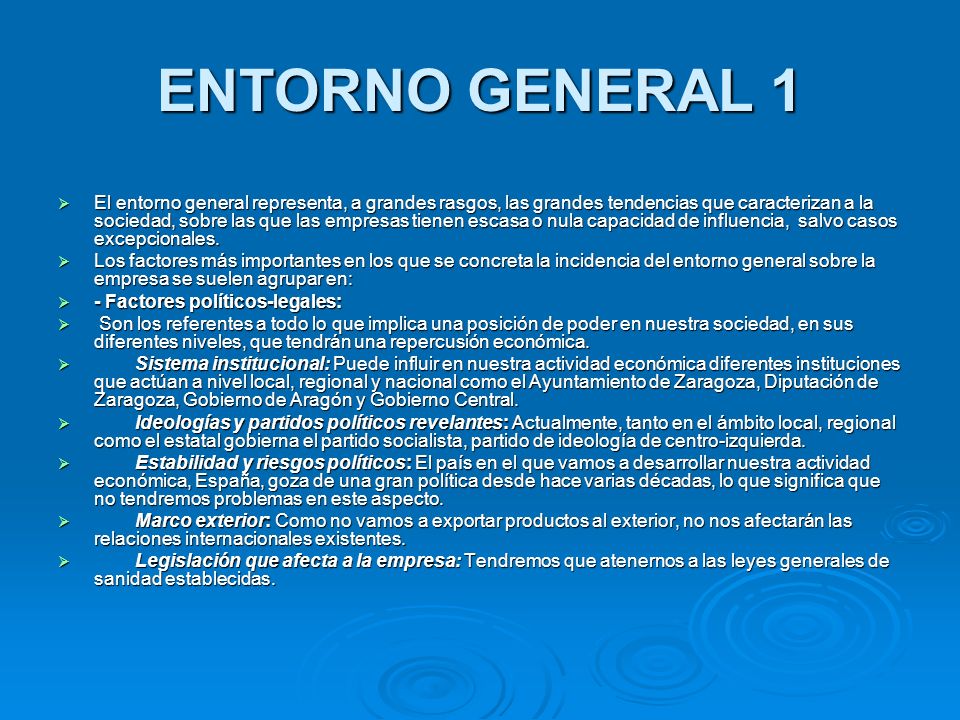The image is a clear, bright-blue PowerPoint slide titled "Entorno General No. 1" with the heading written in white capital letters at the top center. On the bottom right-hand corner, there are artistic illustrations resembling water ripples. The slide is divided into nine bullet points, all in a foreign language, discussing topics such as factories, politics, legal frameworks, institutional systems, ideologies and relevant political parties, political stability and risks, external frameworks, and legislation affecting businesses. Green arrows on the left-hand side point towards these bullet points. The overall image and text are clear, though the specific language is unfamiliar.